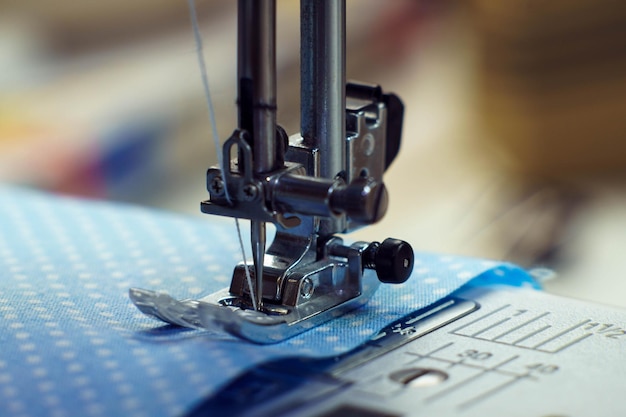The image captures a close-up view of a sewing machine in action, focusing on the intricate part that performs the actual sewing. The machine is threading a piece of blue fabric adorned with white squares or polka dots arranged in angled patterns. Prominently visible is a metallic mechanism with various knobs, metal poles, and black plastic components guiding a piece of thread down to the fabric. A small ruler lies underneath the sewing part, displaying partial measurements with markings such as "1/2 inch," "1 inch," and "40, 30," though the rest is cut off. The sewing area is highly detailed, showing the nib of the metal device inserting the thread into the fabric, held in place by another metallic object. The background is blurred, incorporating hues of yellow, white, blue, red, and beige, keeping the primary focus on the sewing process and the vibrant blue and white fabric.